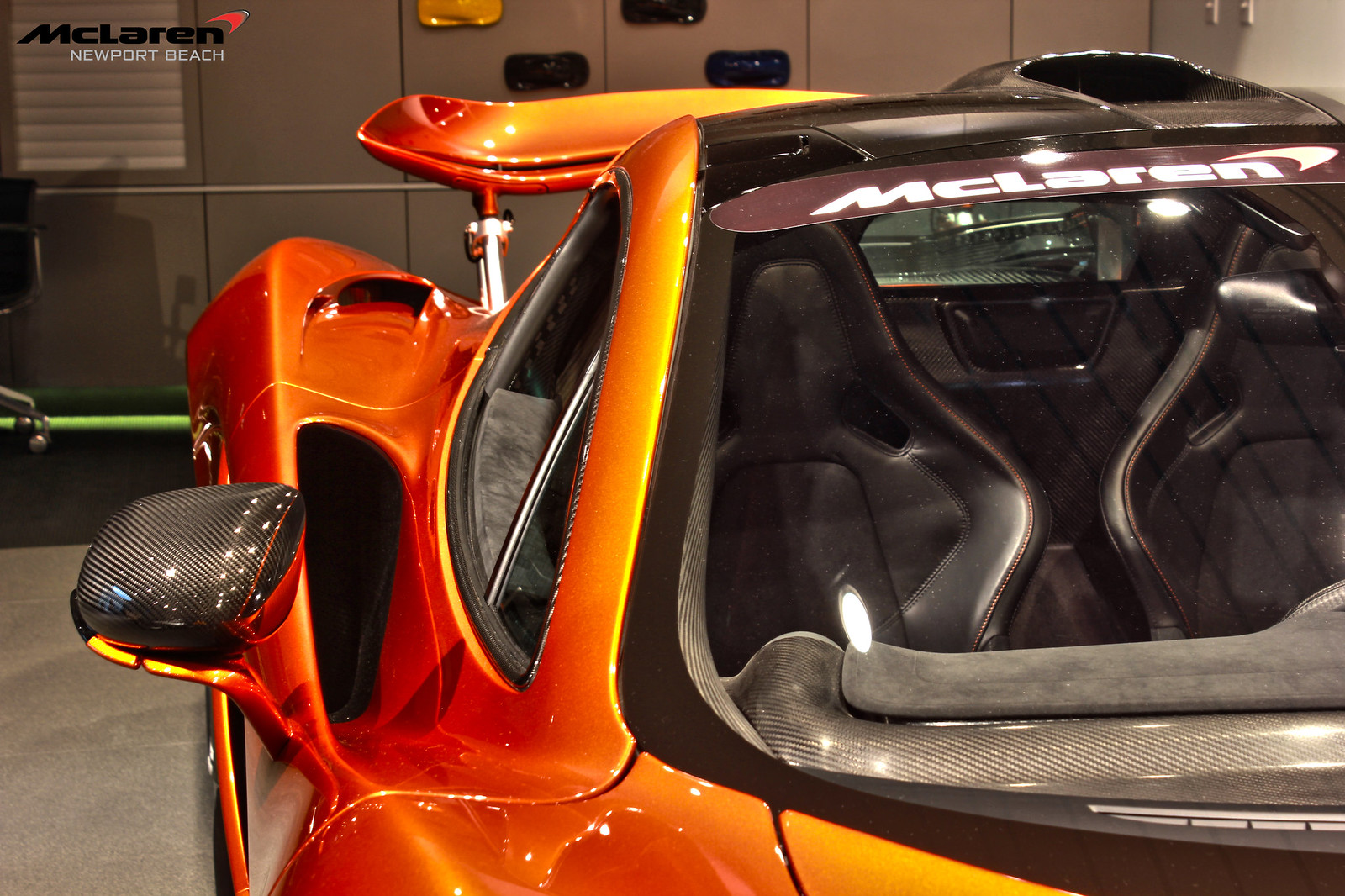The photo captures a vibrant, fiery orange McLaren sports car with a stunning ombre effect that transitions into yellow at certain parts. The image is of the passenger side, viewed from near the front door, revealing the sleek side mirror and side handle. The car is equipped with a prominent rear fin (spoiler) and luxurious black seats visible through the windows. The top of the windshield features a visor that reads "McLaren." The setting appears to be an elegant showroom with a gray-tiled floor, gray walls, and miniature car models displayed in various colors. In the top left corner, a "McLaren Newport Beach" logo is prominently displayed.